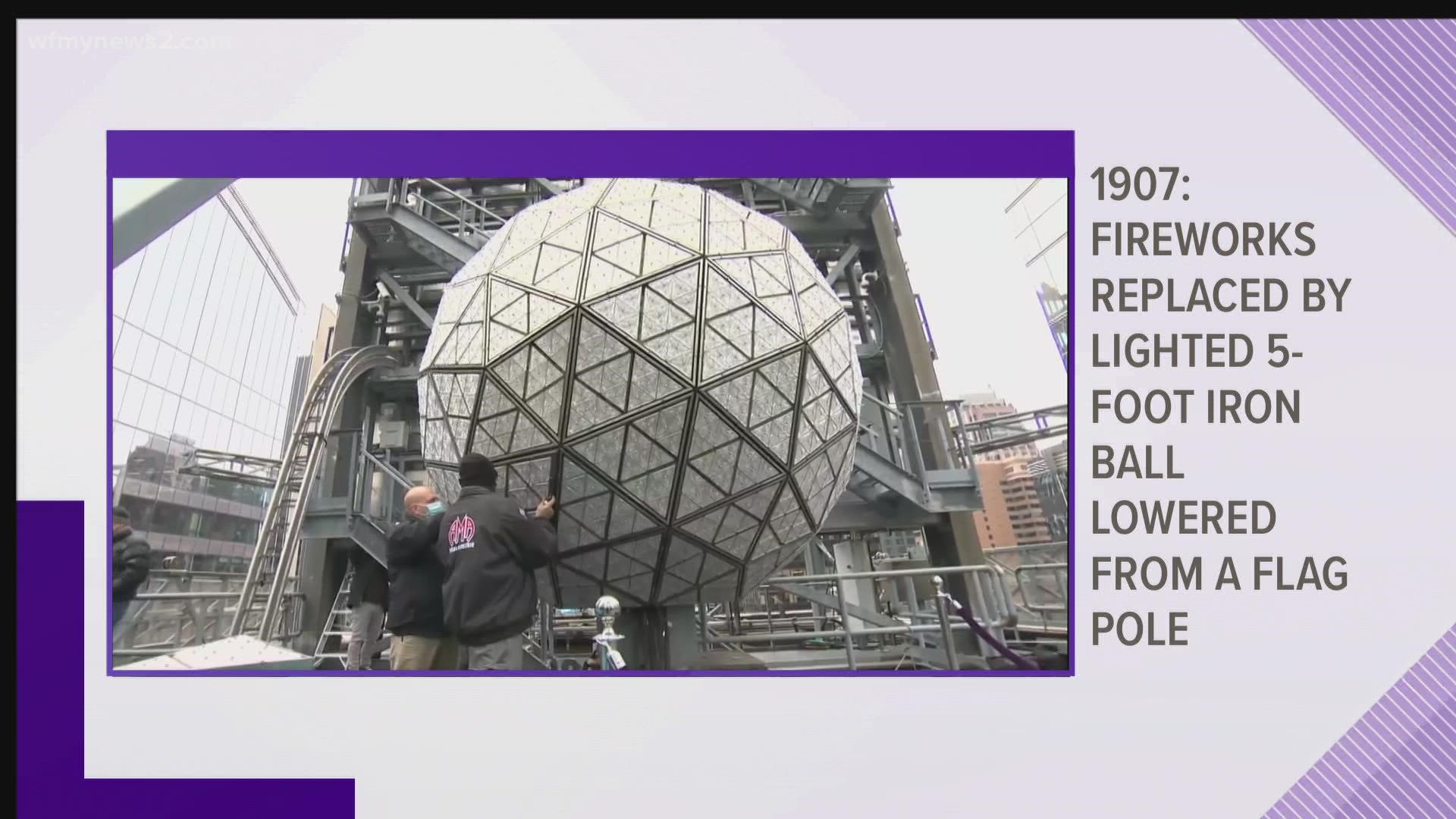The image is a horizontal, rectangular, color photograph set within a PowerPoint slide framed with a light purple background and darker purple designs at the top right and bottom right corners. The photograph, located in the left center of the image and framed in purple, captures a historic New Year's Eve scene from Times Square in New York City, featuring a lighted five-foot iron ball designed to be lowered from a flagpole. Although it is daytime and the ball is not illuminated, two men are present in the lower left corner, inspecting or touching the ball. One man wears a black jacket and a winter hat, facing away from the camera, while the other, who is bald and masked, also wears dark clothing. The ball is part of an iron structure with visible metal railings and stairs, suggesting multiple levels and a ramp ascending from the ground. The background features various buildings on both sides; notably, there is a red brick building in the right corner. To the right side of the photograph, gray text on a light purple background reads, "1907: Fireworks replaced by a lighted five-foot iron ball lowered from a flagpole," indicating the historical context of the scene.